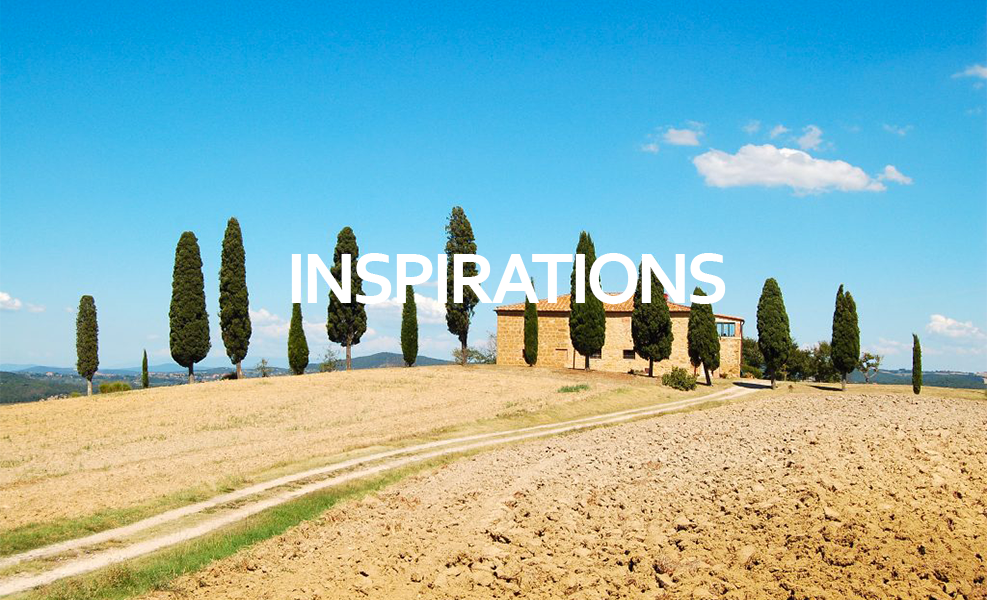The photograph depicts a small, tan brick house with a terracotta roof, nestled in an outdoor rural setting. The foreground features a farm-like landscape with clumpy, brown, and rocky dirt terrain on both sides. A central dirt track or pathway leads directly to the house. Surrounding the house are well-maintained small trees, possibly evergreens, arranged in varying heights. The backdrop includes a swath of open land, giving a sense of a small farmland. A bold white text in all capital letters reading "INSPIRATIONS" is prominently displayed in the center of the image. The sky is a bright blue, dotted with clouds primarily towards the upper right-hand side, indicating a clear day. In the far distance, a faint mountain range is visible, adding to the picturesque and serene rural scene.